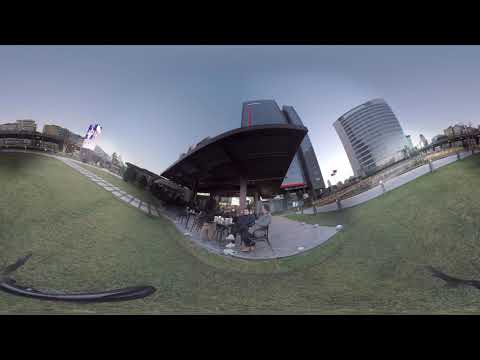This photograph presents an outdoor scene captured with a wide-angle lens, creating a curved, concave effect that gives an optical illusion of a hilly landscape. However, the area in reality is a fairly flat, paved surface. At the center of the image, two people are seated at a small table under an overhanging pavilion, providing shade from the sun. The scene shows additional tables scattered in the background. The photograph is set in an open-air environment that resembles a park or a public square. In the far distance, there are two tall skyscrapers, which could be business complexes or large hotels, framed against the sky. Notably, a neon sign is visible to the left side, positioned in front of some other buildings. The image is bordered by a black frame at the top and bottom, and there is no text within the photograph.